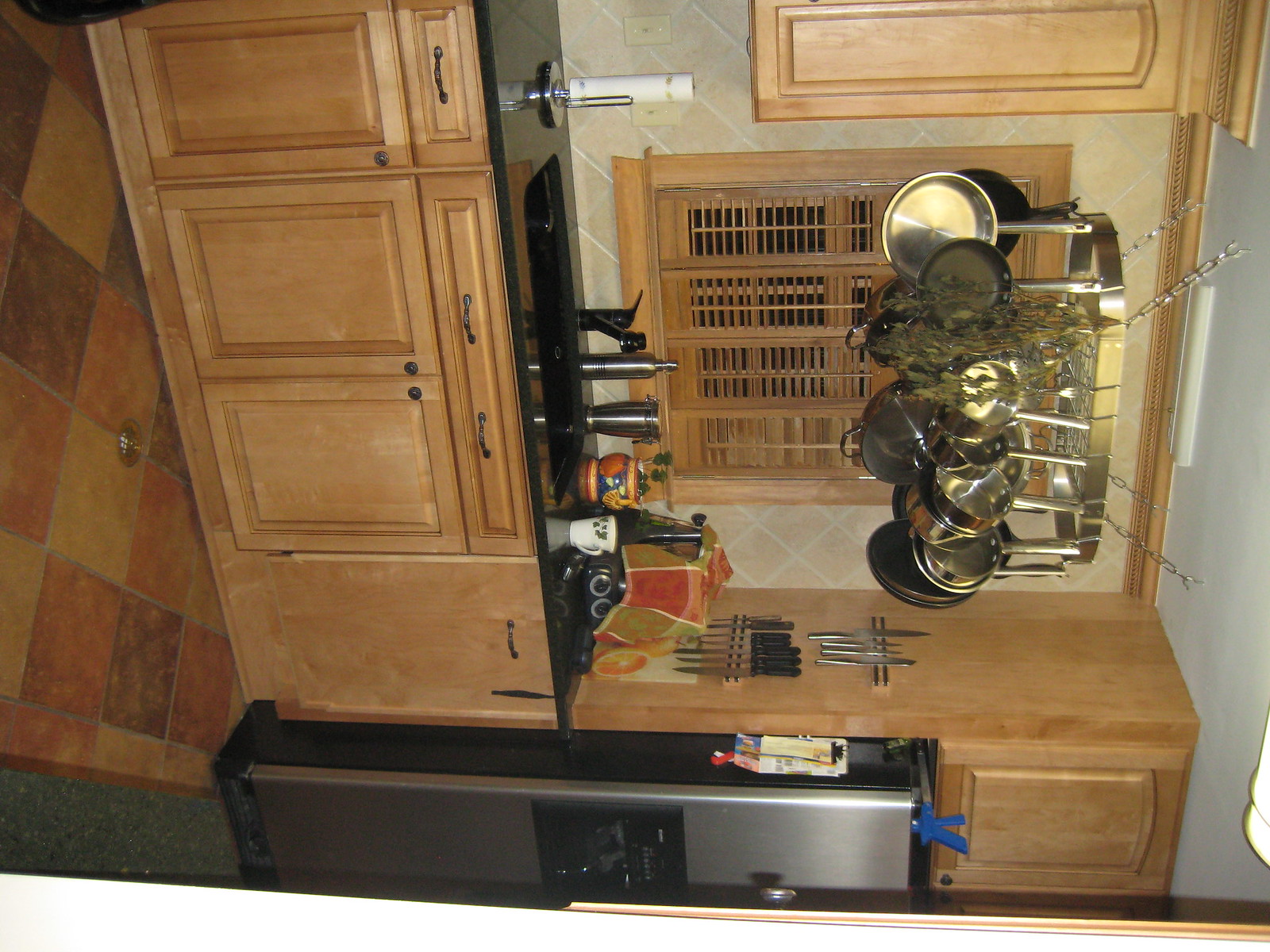In this detailed kitchen scene, the image is initially oriented sideways, so turning it for proper viewing reveals a well-organized space. Centrally above the sink, a ceiling-mounted rack showcases an array of frying pans and pots, underscoring the kitchen's functionality. To the left, a partial view of the cabinet area can be seen, hinting at ample storage. On the right, the refrigerator is seamlessly integrated into the wall with additional cabinets above it, maximizing storage space. Adorning the wall near the refrigerator, a metal magnetic strip elegantly holds various knives, ensuring easy access. On the counter by the sink, a paper towel roll stands ready for use, accompanied by several mugs and a cup containing cleaning sponges, emphasizing practicality. Adjacent to the refrigerator, a coffee maker or a similar kitchen appliance sits discreetly, partially covered by a towel, adding a touch of everyday realism to the scene.